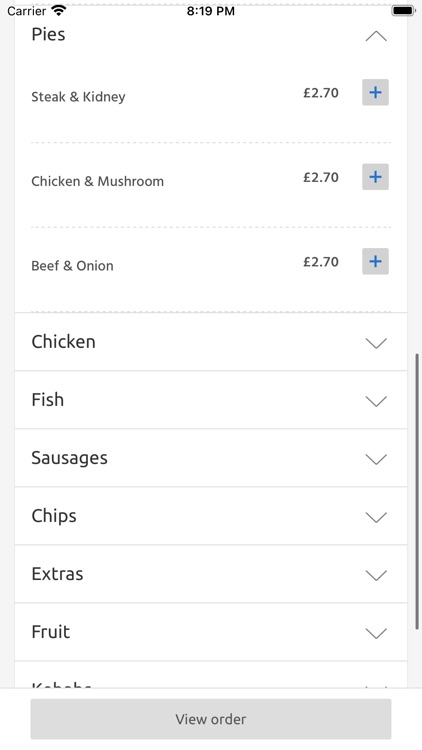Detailed Caption: 

This screenshot from a cell phone features a menu interface. At the very top of the screen, the status bar is visible, showing the Wi-Fi icon, the time "8:19 p.m.", and a fully charged battery icon. The primary content of the screen is a menu listing various food items and their prices. 

At the top of the menu, there is a section labeled "Pies," listing the following items with their corresponding prices:
- Steak and Kidney: £2.70
- Chicken and Mushroom: £2.70
- Beef and Onion: £2.70

Below these listed pies, additional categories are mentioned but not expanded. These categories include:
- Chicken
- Fish
- Sausages
- Chips
- Extras
- Fruit
- Kebabs

At the bottom of the screen, a gray rectangle is present, featuring the text "View Order."

The image is taller than it is wide, presenting a vertical orientation. There are no photographic or illustrative elements, and the image clearly lacks any visual representations of people, animals, plants, buildings, or vehicles.